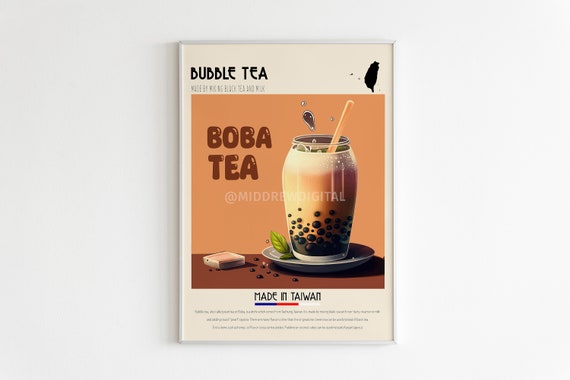This advertisement poster for Bubble Tea, prominently featuring Boba Tea made in Taiwan, is designed with a cream-colored background and a simple white frame, hanging on an off-white wall. The central image showcases a glass of bubble tea with a swirling mix of caramel and milky hues, complemented by a frothy top. Black boba pearls are visible at the bottom of the glass, which is presented on a saucer garnished with a mint sprig. A straw or perhaps a stirring stick protrudes from the glass. Spilled boba pearls and a few dark beans are scattered on the brown table beneath it. Above the image, the text explicitly identifies the drink with phrases "Bubble Tea" and "Boba tea." The statement "Made in Taiwan" is also prominently displayed, underlined subtly by the colors of the Taiwanese flag. Smaller text, unreadable due to its size, rests below the "Made in Taiwan" declaration, adding a touch of intricate detail to the overall composition.